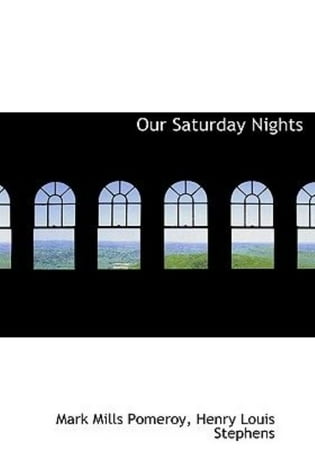The photograph captures the interior of an elegant building, characterized by a series of six arched, uniformly shaped windows that span across the frame. These windows present a stark silhouette against the surrounding darkness of the room, which is pitch black except for the light filtering through them. Through the windows, a picturesque view unfolds, featuring rolling green hills and fields, with a hazy, distant landscape that could be a town, city, or simply more greenery. In the top right corner, white text reads, "Our Saturday Nights," and at the bottom, in a white space, the names Mark Mills Pomeroy, Henry Louis Stevens are inscribed, likely referring to individuals who spend their Saturday nights gazing out these windows.